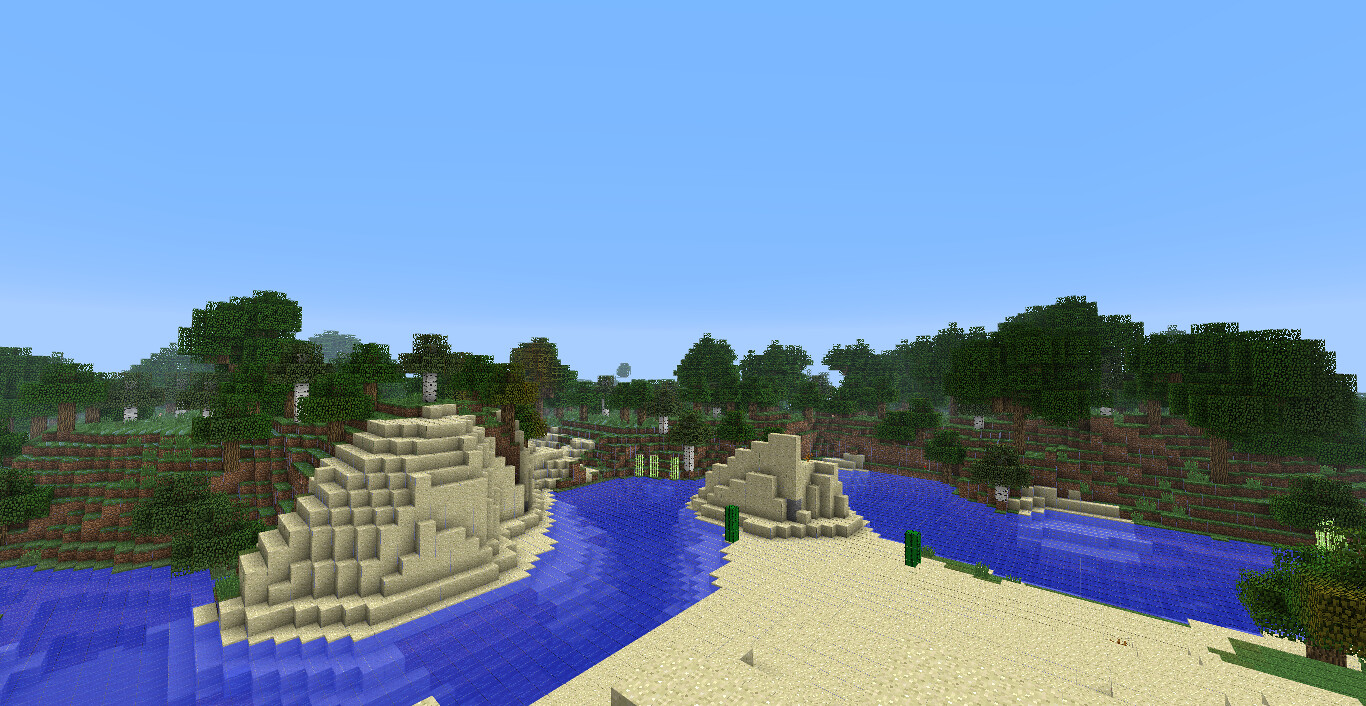This is a screenshot from the game Minecraft, characterized by its distinctive voxel art style. The image showcases a serene scene under a clear, blue sky with no clouds in sight. A dark green tree line stretches across the horizon, featuring the iconic blocky, square textures of the game's foliage.

In the foreground, a sandy beach is depicted with tan-colored sand blocks extending into a deep blue ocean. The underwater sand is visible through the water, creating a gradient of white and lighter blue hues where the two elements meet. The sandy terrain slopes upward to meet grassy blocks at the top of the hill, blending seamlessly into the dense tree line.